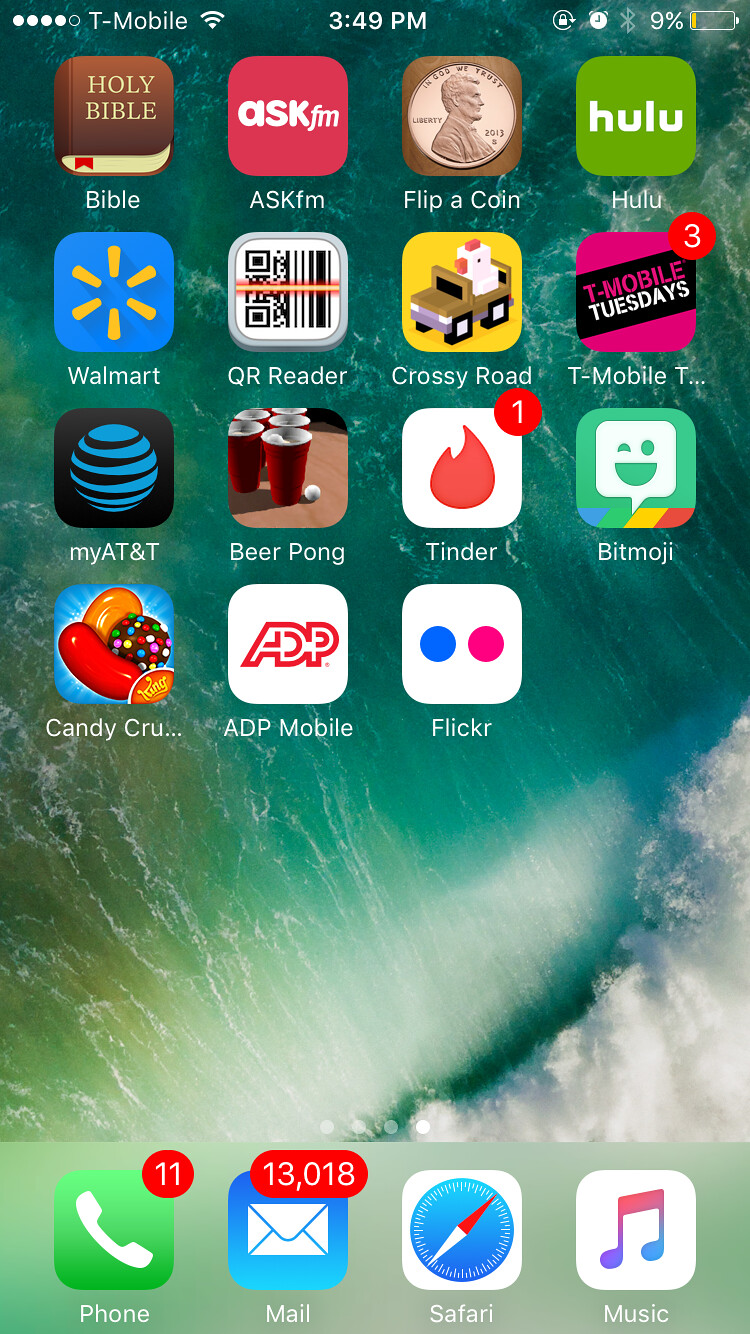The screenshot depicts the fourth page of an iPhone's home screen, identifiable by the fourth dot being highlighted at the bottom. The screen shows a variety of apps arranged from left to right and top to bottom. The apps include: Bible, Ask.fm, Flip A Coin, Hulu, Walmart, QR Reader, Crossy Road, T-Mobile, My AT&T, Beer Pong, Tinder, Bitmoji, Candy Crush, ADP Mobile, and Flickr. Notifications are visible for three apps: three notifications for T-Mobile, one for Tinder, and the Phone app in the home row shows 11 notifications. Additionally, the Mail app displays an overwhelming 13,018 notifications. The home row also includes Safari and the Music app. 

The background is a green wave, likely a default image provided by Apple. The status bar indicates the phone carrier is T-Mobile, with full signal strength denoted by four dots, active Wi-Fi, and it being 3:49 p.m. Additional icons show that the auto-rotate mode is locked, the alarm is active, Bluetooth is enabled, and the phone battery is critically low at 9%.